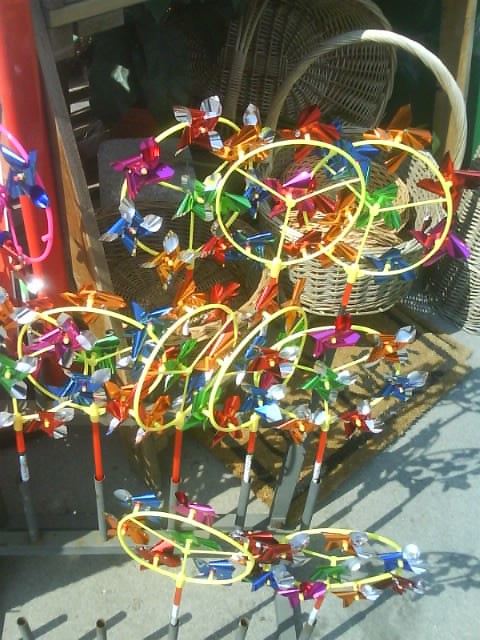In this outdoor rectangular portrait image, there is an array of colorful pinwheels displayed in front of a gray-paved driveway. The pinwheels are mounted on two long metal stands with narrow vertical tubes. Most of these tubes feature pinwheels, while a few remain empty. The pinwheels have distinctive red handles which are longer than their circular tops. Each pinwheel top consists of a large yellow circle supported by three triangular bars in a peace sign shape. These circles are adorned with cheap-looking plastic ribbons shaped like flowers in various colors such as purple, silver, red, blue, and green, suggesting the objects might spin in the wind.

In the foreground, there is a systematic arrangement of nine pinwheels in three rows: two at the bottom, four in the middle, and three at the top, while on the left, there appears to be an additional pink-circled pinwheel. The vivid pinwheels cast shadows on the pavement below. 

In the background, an outdoor storage area houses several large, empty wicker baskets, some tilted so that their openings are visible. This detailed scene appears to be part of a vendor's display, showcasing these vibrant wind-catching devices.